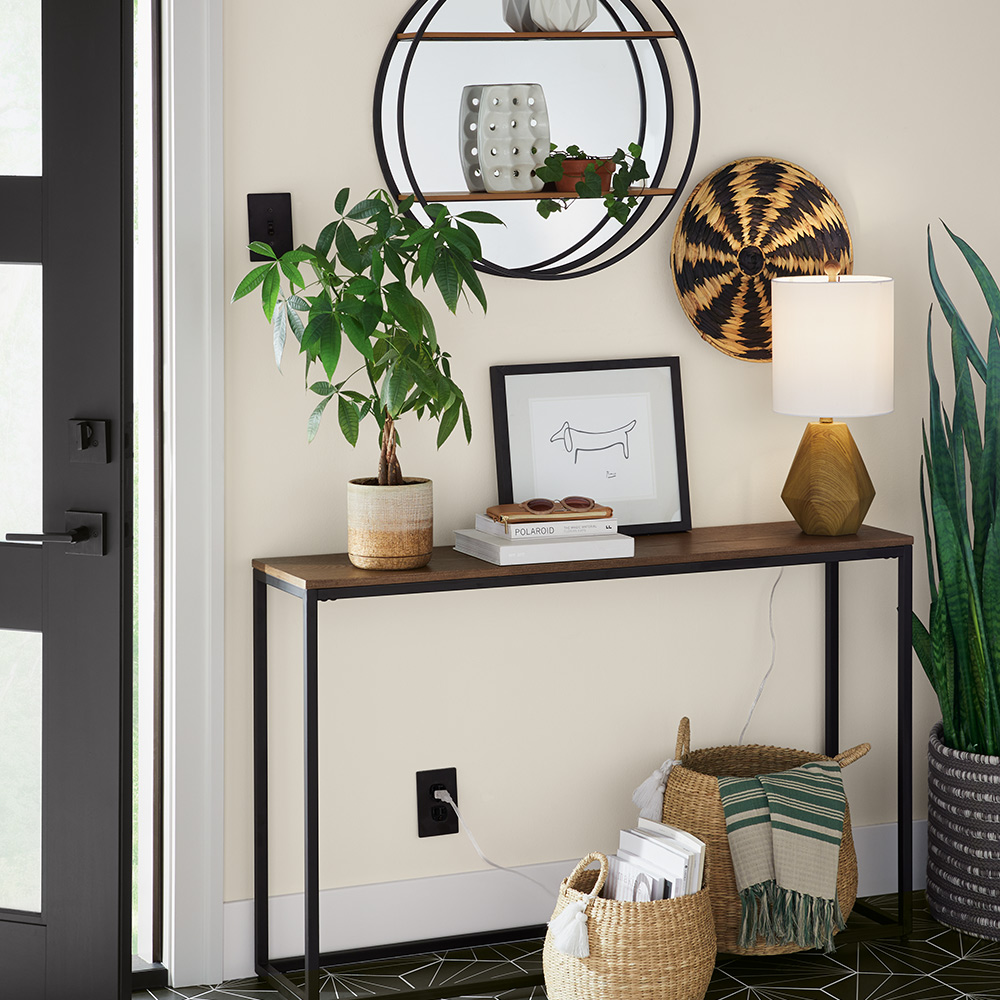The image depicts a cozy interior scene focused on a white wall adorned with various items. On the left side of the wall, there is an open black-framed door with a white glass panel. Above, a circular metal frame with two levels serves as a shelf, holding two white objects and some green plants. Just below this shelf, a brown wooden bench is positioned, featuring a white and brown pot with green plants on its left side. A simple black-line drawing of a dog in a black frame is also visible.

In front of the wall, there is a small brown desk table with black legs. On the table are several items: a green plant, a framed picture of a dog drawing, a pair of glasses, and some books. To the right of the drawing sits a yellowish-gold lamp with a white round lampshade. An outlet is visible to the left of the table, with a cord running through it. On the floor beneath the table, two wicker baskets are stored—one contains a green striped blanket and the other holds books and envelopes. Further to the right, there is a tall snake plant with thin green leaves in a gray striped basket. The area exudes a warm, lived-in charm, accentuated by a black-tiled floor.